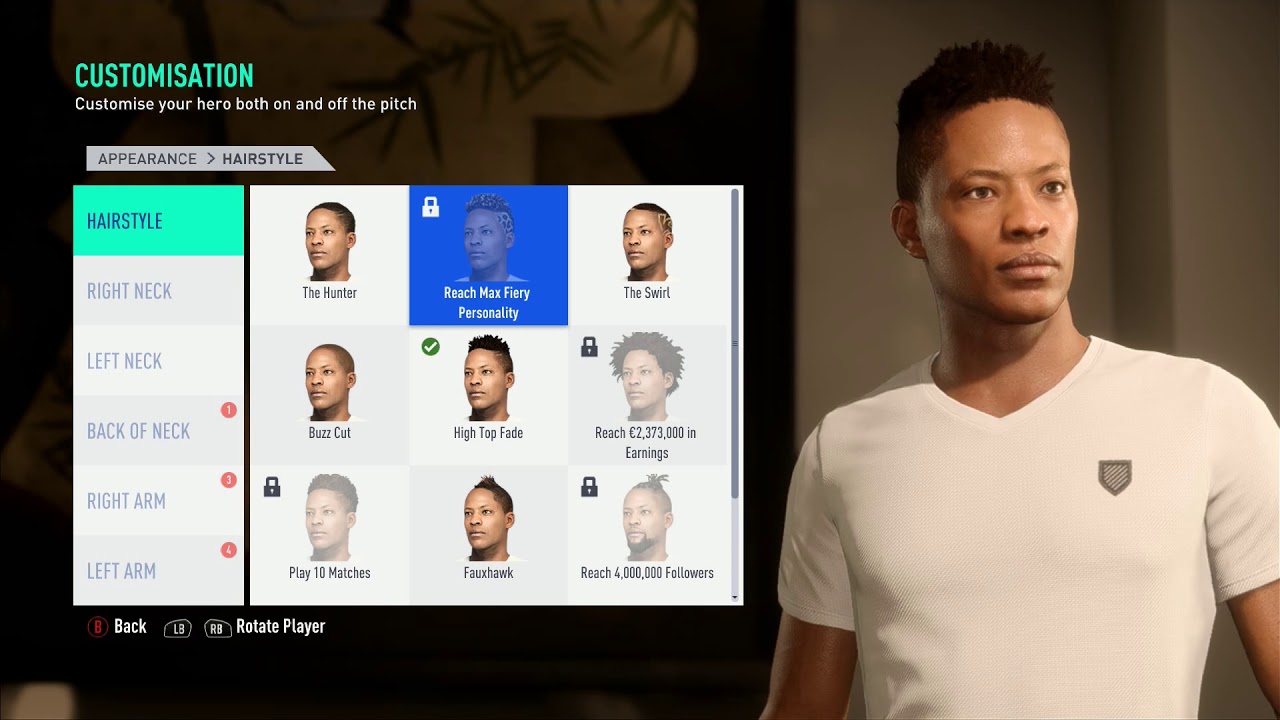The image is a screenshot from a photorealistic soccer video game, featuring the character customization menu. Dominating the right side of the screen is a detailed depiction of the character being customized - a Black man in his late 20s to early 30s. His hair is styled in a high top fade, with a couple of inches of length on top and closely buzzed sides. He is dressed in a white t-shirt adorned with a silver shield logo on the left side of his chest, and his gaze is directed towards the right.

To the left of the character, the customization menu is prominently displayed. The light green text at the top reads "Customization," with a subheader stating, "Customize your hero both on and off the pitch." This indicates that the game involves soccer and allows for character personalization in various contexts. The current section being viewed is "Appearance," specifically the "Hairstyle" category. The high top fade is the selected hairstyle, marked by a green checkmark. Additional hairstyles are seen, but some are locked, requiring either in-game purchasing or reaching a certain level to unlock those options.